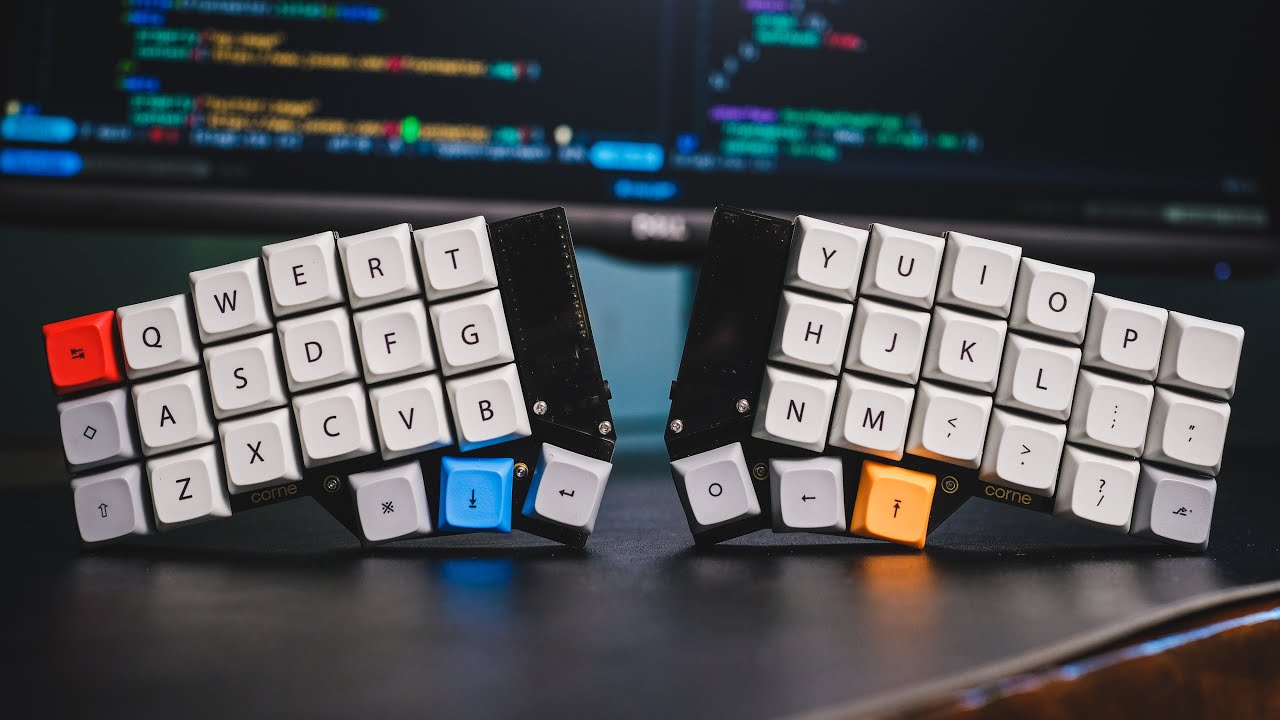The photograph captures a custom-built split keyboard prominently positioned on a plain gray desktop. The keyboard is divided into two separate halves to facilitate ergonomic hand placement. Each half is standing upright, showcasing the intricate key layout. The keys are predominantly beige or off-white with black lettering, accented by a few distinctively colored keys: a bright red key on the top left of the left half, a blue key with a down arrow, and an orange key on the right half. In the background, a computer monitor displays colorful coding text in an array of colors including orange, blue, red, green, purple, and teal, against a black screen. Despite the blur making the text unreadable, the colorful script creates an engaging and vibrant backdrop to the keyboard setup. The entire image is front and center, highlighting the unique design of the keyboard without a space bar, making it an integral part of a well-organized and visually appealing workspace.